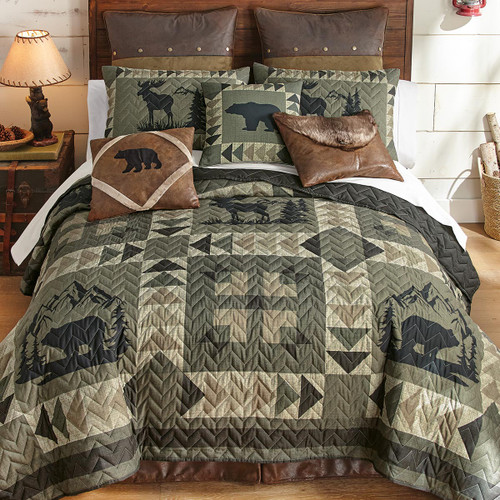This photograph captures a cozy bedroom with a rustic, cabin-like aesthetic. The main focus is the bed, seen slightly from above, featuring a square wooden headboard. The bed is adorned with a variety of pillows, including brown leather-like ones and decorative green ones showcasing animal designs such as bears, moose, and deer, as well as trees and mountain symbols. The comforter is gray and white with triangle patterns and silhouettes of black bears and moose, matching the pillow shams at the top of the bed. There is a sturdy green quilt layered over the bed. Nearby, a nightstand resembling a treasure chest holds a lit lamp with a white lampshade, its base mimicking a wooden tree branch. The room has hardwood floors and white walls made of large, brick-like material.